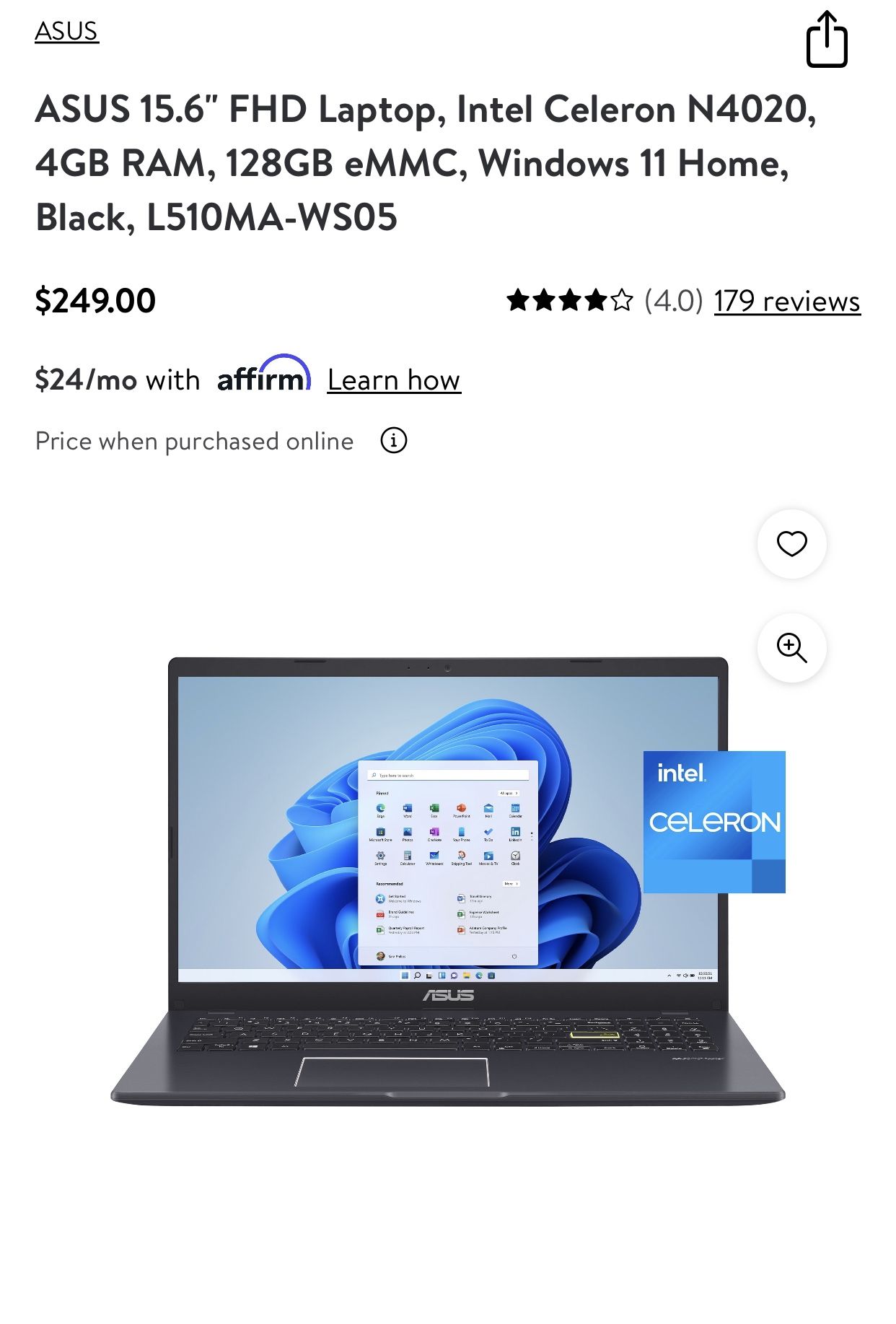The image is an advertisement for a computer. At the top left corner, in black font, it prominently features "ASUS" underlined in large letters. Below this, in even larger print, it states "ASUS 15.6 inch FHD Laptop Intel CELERON N4020," followed by "4GB RAM, 128GB eMMC, Windows 11 Home, Black, L510MA-WS06". Directly beneath this description, the price is listed as "$249" with a preceding dollar sign. Additionally, the product has achieved a 4-star rating out of 5, based on 179 reviews. Below the price, it mentions a financing option: "$24/mo with Affirm," followed by an underlined "Learn how." It also specifies that this is the price when purchased online.

The central image showcases the laptop itself, which is black, with the screen open. The display shows a blue, swirly background design, overlaid with a box containing various computer icons. To the right of the laptop, there's a blue label that highlights "Intel CELERON".